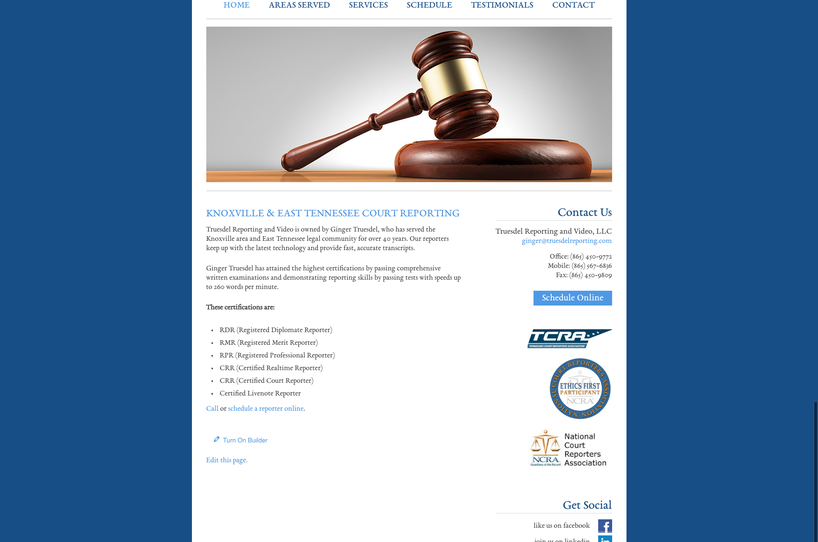The photograph showcases a web page design predominantly featuring a white and blue color scheme. Along the sides, there are blue panels framing the central white content area. At the top of the page, navigation tabs are visible: "Home" is highlighted in light blue, while "Areas Served," "Services," "Schedule," "Testimonials," and "Contact" are displayed in dark blue.

Beneath the navigation bar is a graphic illustration of a gavel, complete with a round wooden base and a handle featuring the round striking surface. Just below this image, the text "Knoxville and East Tennessee Court Reporting" is prominently displayed.

The page includes a "Contact Us" section that lists phone numbers and provides a hyperlink leading to another web page. Additionally, there is a prominent "Schedule Online" button for convenience. 

Supportive affiliations and mentions such as TCRA (Tennessee Court Reporters Association), Ethics First Participant, and the National Court Reporters Association are highlighted, alongside social media icons for Facebook and LinkedIn.